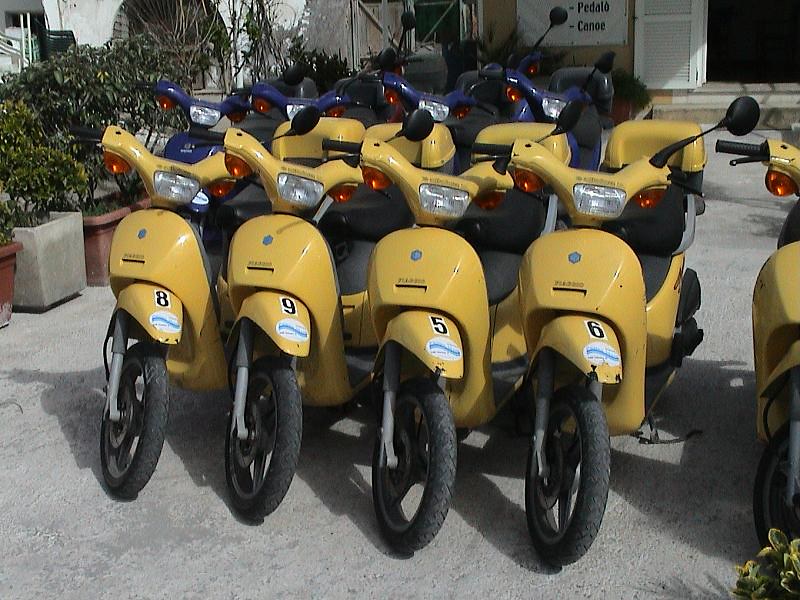This color photograph captures a vibrant scene outside a rental shop, likely in Spain, given the Spanish text. The image focuses on two rows of small motorbikes, each meticulously lined up. At the center, four yellow Vespa-type scooters dominate the front row, their fenders numbered 8, 9, 5, and 6. A partially visible yellow scooter appears on the right side. Behind the yellow scooters, four blue ones of the same style stand in formation. Each scooter features a sticker, presumably showcasing the rental place's logo. In the background, there's a white cement wall with a small window and shutters visible in the upper right-hand corner. A sign on the wall advertises "Pedal Canoe" rentals. To the left of the scooters, several potted plants with lush green foliage add a touch of nature to the scene. Some of the pots are brown, while others are grey. The scooters and their surroundings suggest a lively, well-maintained area for tourists and locals to rent bikes and other equipment.